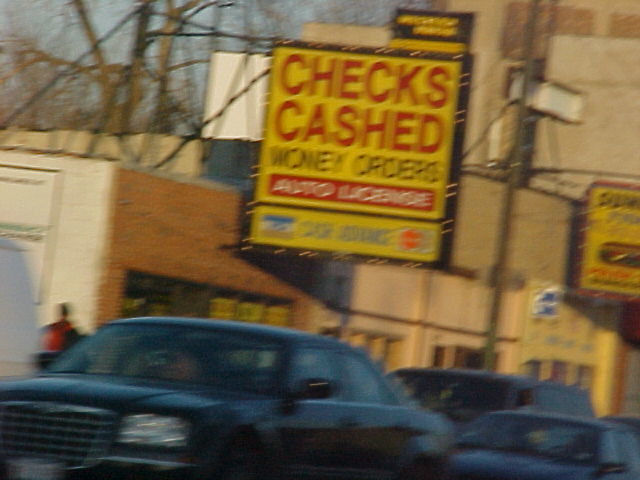The image captures a slightly blurry, low-quality photograph of a city street scene featuring a check cashing establishment. The street is lined with three dark-colored cars, possibly black, all positioned toward the left side of the photograph. The centerpiece of the image is a small, worn-looking brick building on the right-hand side, partially painted white.

The building prominently displays a large yellow sign with bold black and red letters, reading "Western Union" at the top, followed by "Checks Cashed" in red, "Money Orders" in black, and "Auto License" in a red oval with white writing. Though slightly blurry, the sign also features Visa and MasterCard symbols on either side. 

In the background, the upper part of the photo shows old and worn buildings to the left and trees peeking above the structures to the right, suggesting a less affluent area. Another large yellow sign is visible two doors down but is too blurry to discern any details. A man stands in front of the check cashing store, though his features are indistinct due to the photo's low quality and motion blur.